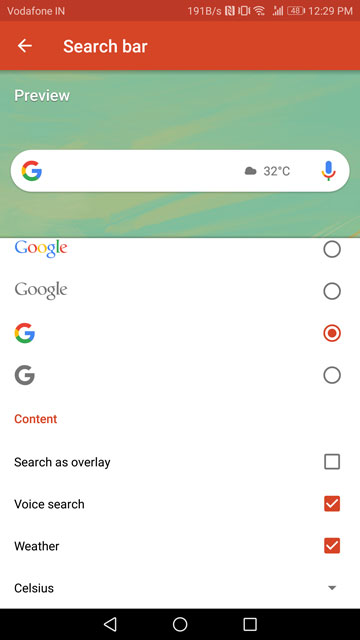The image depicts a user interface commonly found on websites or applications dedicated to customization. Dominating the top portion is a banner in a reddish-orange hue labeled "Search Bar." Directly beneath this banner, positioned towards the left, is the word "Preview." Centered within this section is a mockup of a Google search bar.

On the left end of the search bar, the familiar Google "G" icon is prominently displayed. On the opposite end, there's a weather icon showing a gray cloud, accompanied by a temperature reading of 32°C. At the far right, the search bar concludes with an icon representing a microphone, signaling the option for voice search functionality.